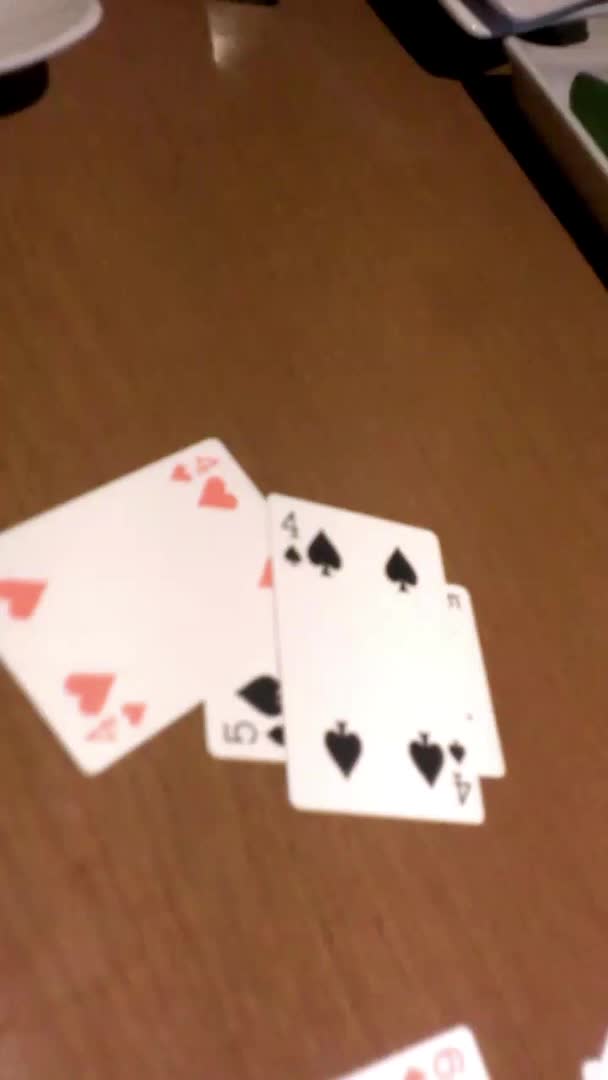A slightly out-of-focus photograph captures a medium brown wood grain tabletop. The image prominently features portions of five playing cards in various positions, suggesting motion at the time of capture. At the base, just the tip of a card showing the number six is visible. In the lower right corner, the tip of another card emerges. Central to the composition, three playing cards are scattered in a stacked, overlapping pattern. The base card, the five of spades, appears horizontally. Angled above it is the four of hearts, and at the top of the pile, most vertically positioned, is the four of spades. To the top and top right of the image, indistinct items that resemble dishware or meal-serving pieces can be seen, adding to the casual, everyday ambiance of the scene.